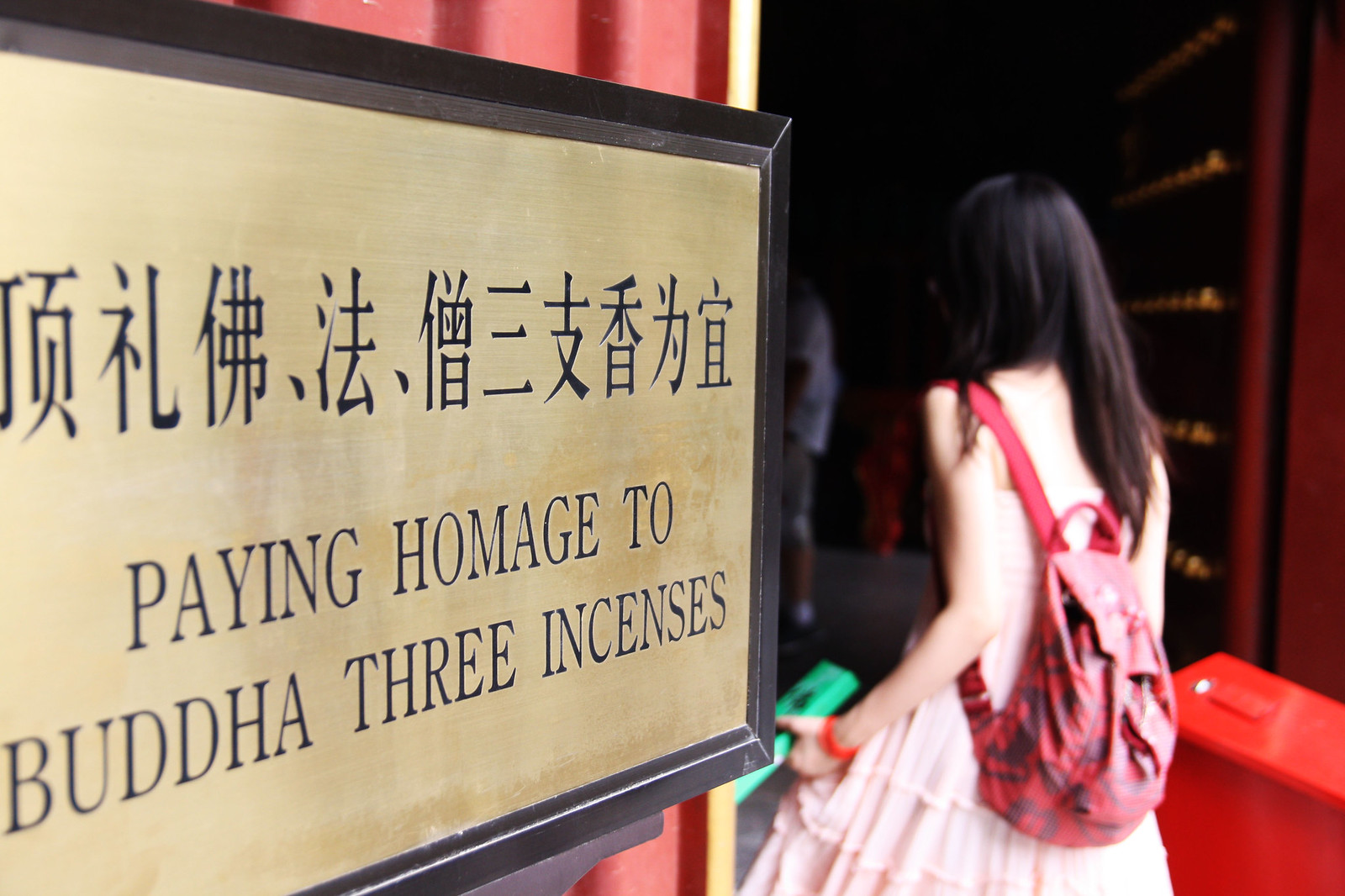On the left side of the image, there is an angled rectangular object, creating a perspective effect that makes it appear smaller as it approaches the center. This rectangular object is bordered by a black strip and has a metallic gold-colored interior. At the top of the rectangle, a line of characters written in a foreign language is visible, accompanied by English text beneath them. The English text, in black letters, reads, "Paying homage to Buddha - Three Incenses." 

On the right side of the image, a girl is walking into a building, although she is out of focus. She has long black hair that extends to between her shoulder blades and is wearing a pink dress. The girl carries a darker pink backpack and holds a green book in her left hand. An orange-colored bracelet adorns her left wrist. In the bottom right corner of the image, there is a brightly colored orange box with a white spot on its top.